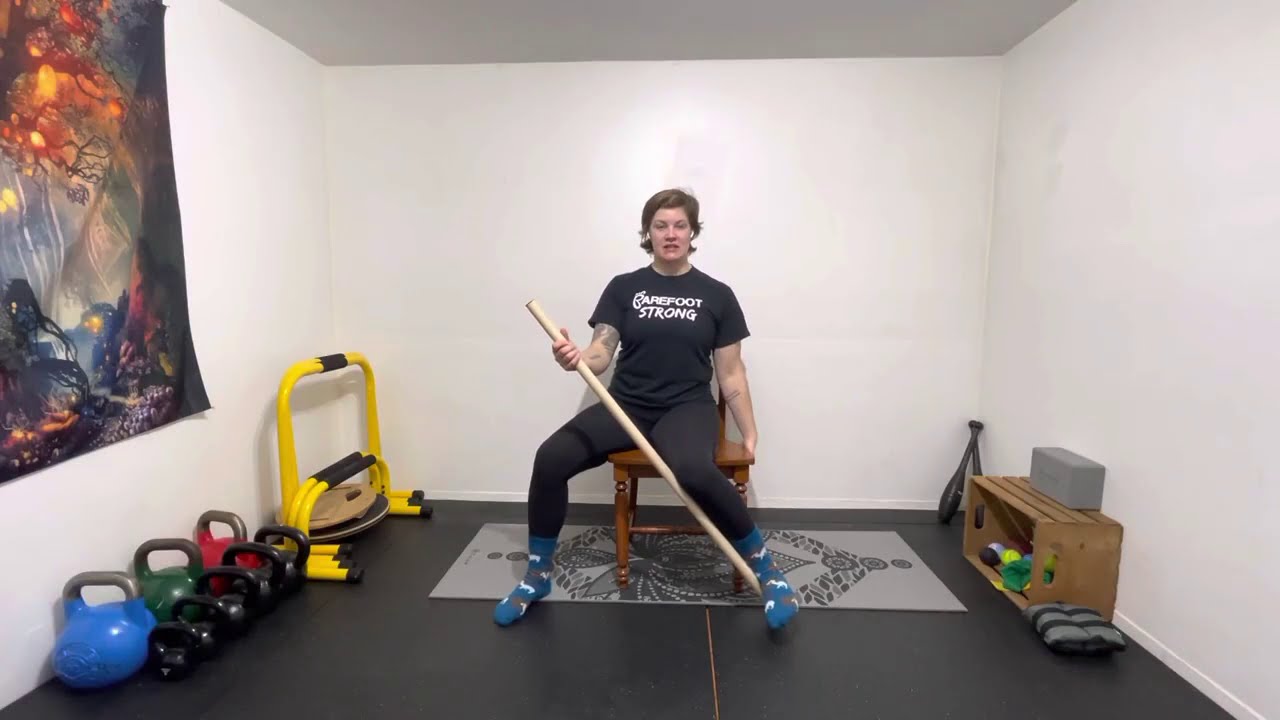The image is a screen grab from a fitness instruction video featuring a young woman sitting on a wooden chair placed on a gray and black patterned yoga mat. The room is set up as a small gym, with white walls and minimal decorations, except for a poster on the left wall depicting a fantasy forest scene with dark and light patches. The woman is dressed in a black shirt with white lettering that reads "Barefoot Strong," black pants, and blue socks with white and brown designs. She is wearing white AirPods and has tattoos on her right arm. In her right hand, she holds a wooden pole, positioned diagonally from her right hand down to her left foot. The room is equipped with various fitness apparatuses, including several colorful kettlebells on the left—a large blue one, slightly smaller green and red ones, and four smaller black ones. There are also parallettes and grips used for dips and handstands, along with a wooden crate containing a yoga block and various pads.